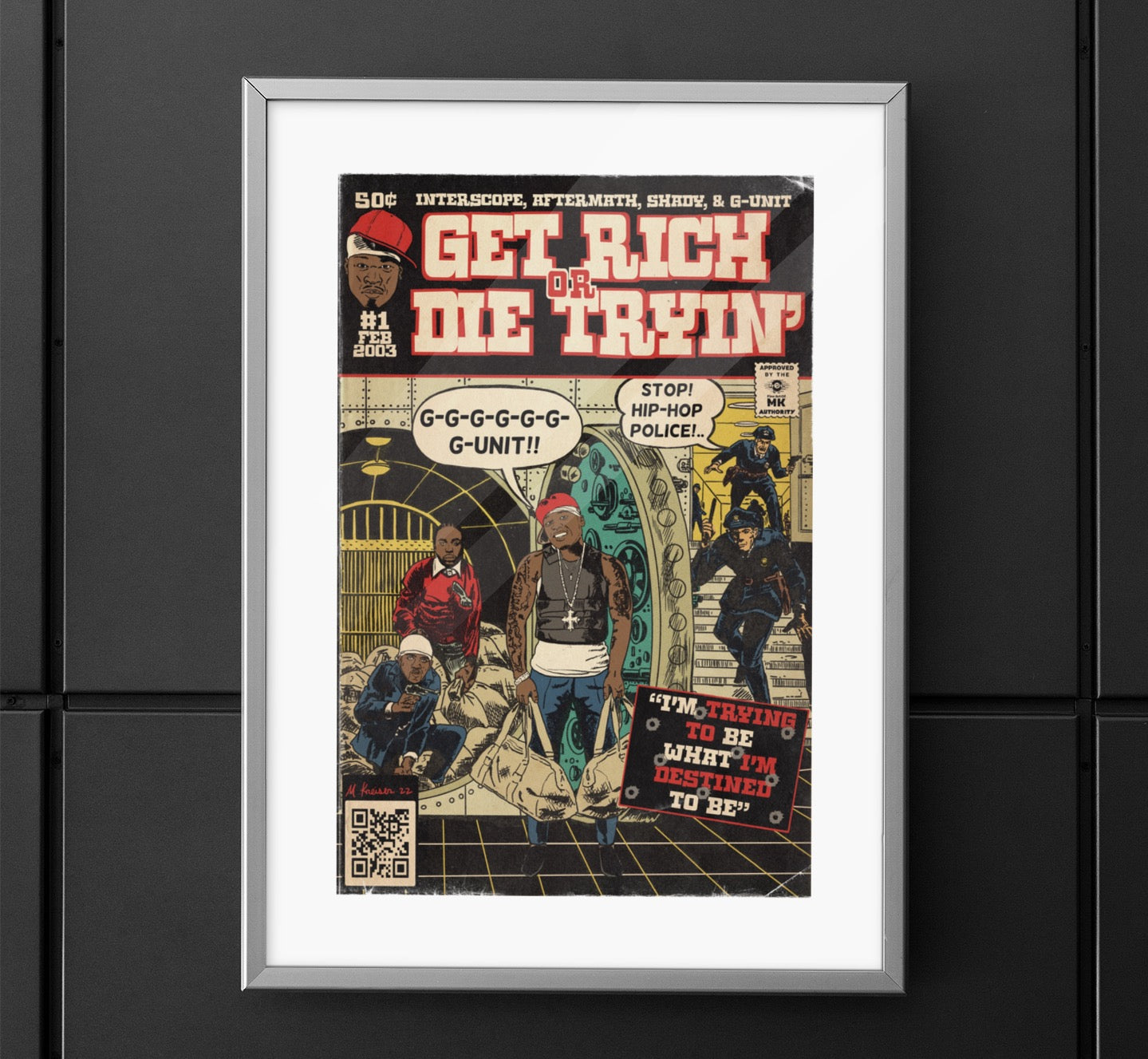The image is a photograph of a framed comic book cover titled "Get Rich or Die Trying," featuring rapper 50 Cent. The frame is a thin silver metal rectangle, slightly larger than the comic book, mounted on a white background against what appears to be a black tiled wall. At the top of the cover, the title is in bold lettering against a black background, with names including "Interscope, Aftermath, Shady, and G-Unit" prominently displayed.

The comic book cover itself is vividly colored and portrays an African-American man, resembling 50 Cent, in a bank heist scenario. He is depicted wearing a red baseball cap, a white handkerchief around his forehead, a black vest exposing his tattoo-covered arms, blue jeans, and a cross necklace. He is holding two money bags, one in each hand, standing in front of a gray bank vault with its door open, revealing stacks of money inside.

To the left of the main character, two figures, seemingly his accomplices, are dressed in red and blue attire. On the right, two police officers in blue uniforms are descending a staircase, shouting, "Stop! Hip-Hop Police!" The main character’s speech bubble reads, "G-G-G-G-G-G-G-Unit."

In the upper left corner, the comic book is marked as issue number one, dated February 2003. At the bottom of the cover, a small black box contains the text, "I'm trying to be what I'm destined to be," reflecting the ambition and thematic essence of the character and, presumably, 50 Cent’s own life.